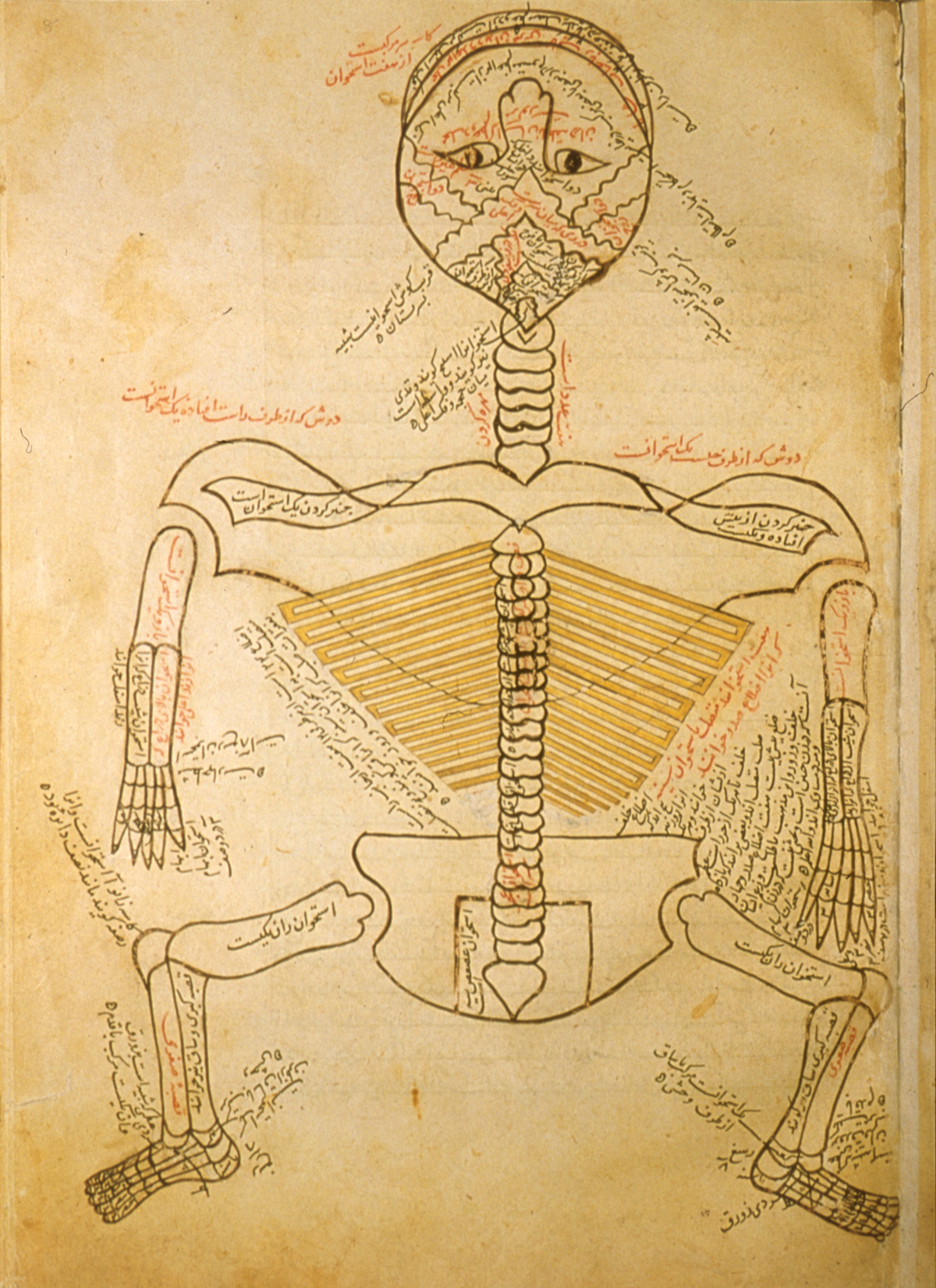This image depicts an intriguing anatomical drawing sketched on an old, oxidized parchment that appears beige and brown, giving it an aged and stained look. The artwork, rendered in brown ink, prominently features a human skeleton with distinctive details. The head at the top of the drawing showcases an inverted face with only eyes and a nose, accentuated by squiggly marks. The body comprises a detailed portrayal of the skeleton, including the spinal cord depicted as a series of circular loops stacked upon each other. The shoulders are broad and rounded, extending into arms configured in a bent "L" shape. The legs are similarly angled at the knees, with feet positioned outward. Surrounding the anatomical structure, various text elements are meticulously placed around different body parts, written in a non-English script that resembles Middle Eastern languages, potentially Hindi, Persian, or Georgian. This unique and somewhat abstract representation of the human skeletal structure, coupled with the mysterious foreign inscriptions, adds a layer of enigmatic character to the drawing.